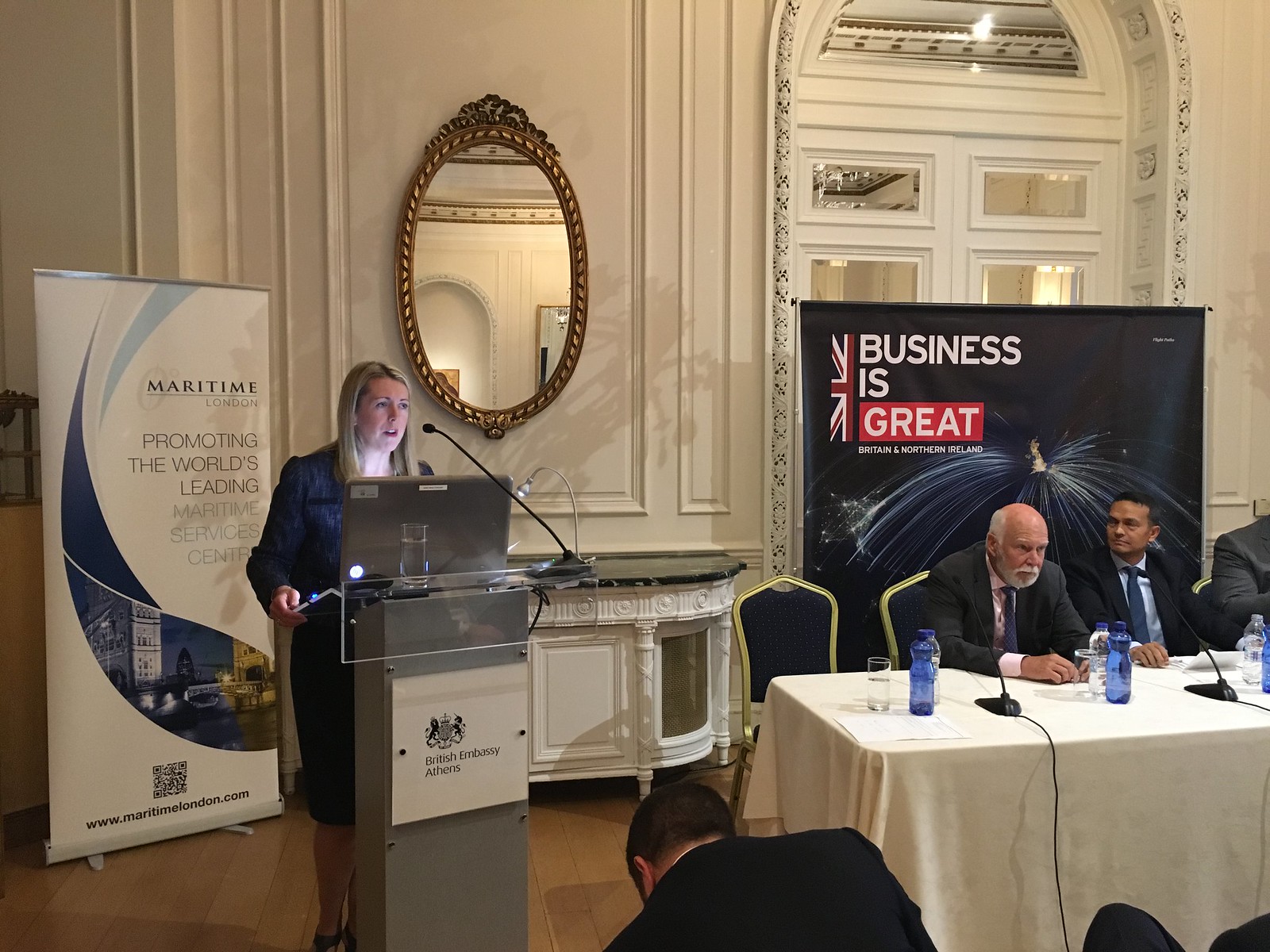The image showcases an ornate interior of a building, resembling an elegant ballroom, where a conference is taking place. At the forefront, a blonde woman in a blue dress stands behind a gray podium emblazoned with "British Embassy, Athens." She speaks into a relatively high-positioned microphone, with a computer screen visible just below it. The walls are intricate and structured, featuring decorative rectangles and a prominent doorway with glass panes and a sign displaying the United Kingdom flag and the phrase "Business is Great," accentuated with firework-like streaks.

To the right of the podium, three men in suits are seated at a white table, equipped with microphones and water bottles. The first man is bald with a white beard and mustache, the second appears to be of South Asian descent in a blue tie, white shirt, and black suit, and only the shoulder of the third man, dressed in a gray suit, is visible. The room’s flooring is a warm brown wood, and behind the podium, a poster reads "Maritime London, promoting the world's leading Maritime Service Center," against a white background with nautical imagery.

A gold-framed mirror to the left of the woman reflects the room's grandeur, and beside it, a chair likely vacated by the woman now speaking. Despite the setting's elegance, the atmosphere is one of focused attention as the audience listens intently to the presentation.